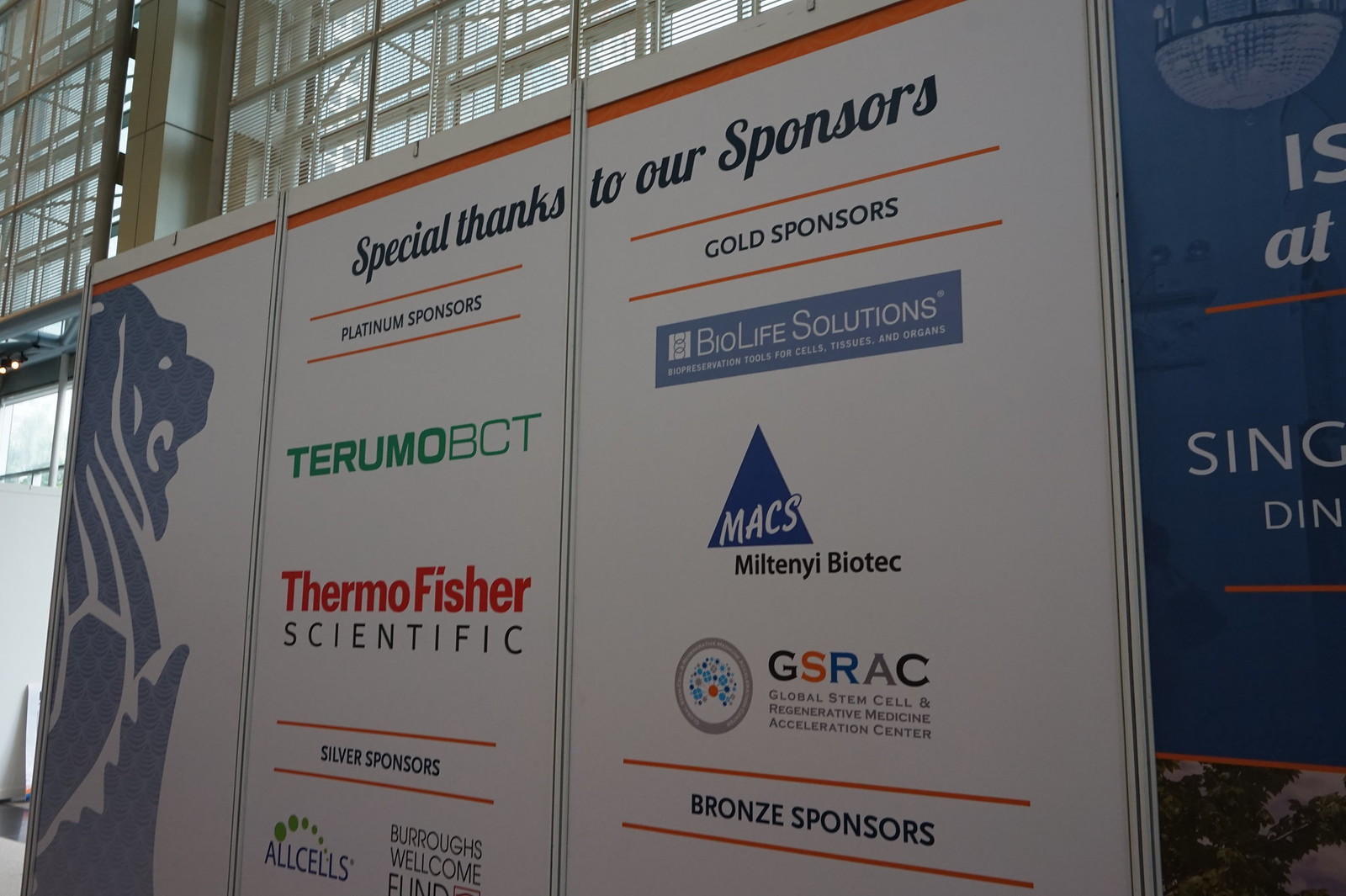This photograph features a large sponsorship board, prominently placed against an indoor wall composed of a series of glass panels and screens with white borders resembling window frames. The wall, visible in the upper left corner and extending to the right, accentuates the modern interior design of the building. The board itself has a white background segmented into three vertical sections. 

On the left section, a blue lion cutout catches the eye, and beneath it, 'Platinum Sponsors' is written in bold black letters. Listed here are company names such as Terium OBCT and Thermo Fisher Scientific. The middle section features additional sponsor names and categories, including Silver Sponsors like Wholesale and Burrows Welcome Fund. 

The rightmost section, highlighted with a touch of blue, displays 'Gold Sponsors' including BioLife Solutions, MaxMittany Biotech, and GSRAC. However, the names of the Bronze Sponsors fade out of view, and their details are not fully captured in the image. The top of the board prominently reads "Special Thanks to Our Sponsors," acknowledging the contributions of these various entities. Above and around the board, the architectural details of the glass panels and possibly metallic nets contribute to the sophisticated ambiance, allowing glimpses of the sky above.